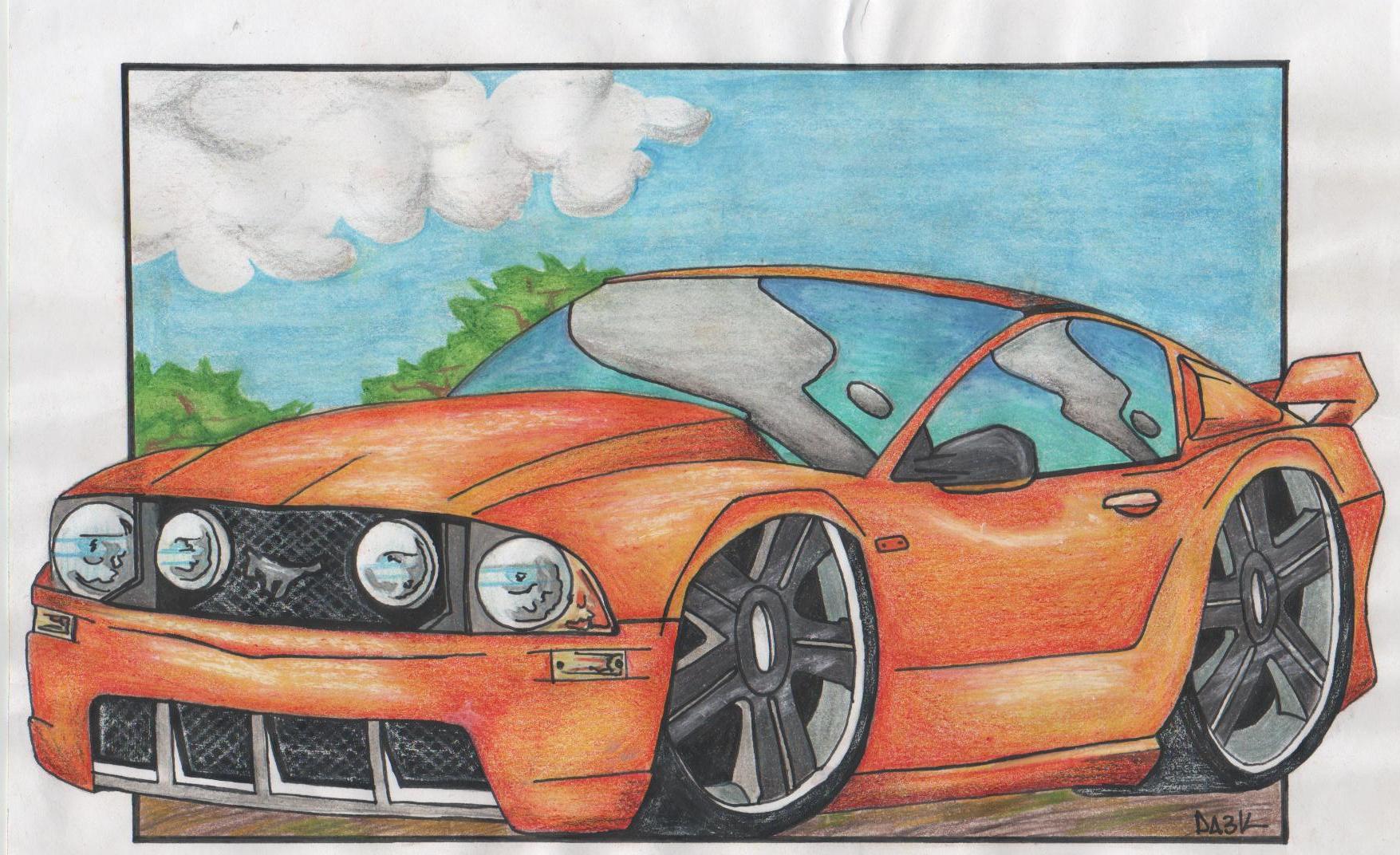The image showcases a meticulously colored pencil or crayon drawing of a sports car resembling a Mustang. The car's vibrant orange paint is skillfully shaded with lighter and darker hues, accentuated by white highlights that add depth to the vehicle's body. Prominently positioned on the left side of the drawing, the front of the car features four circular headlights, gleaming white with subtle gray shades. The centrally situated grille, depicted in a black and gray grid pattern, houses a silver Mustang logo. The windshield and windows reflect a light blue sky adorned with clouds, contributing to a polished and realistic appearance. Above the car, a serene light blue sky with fluffy white clouds enhances the background. The drawing is executed on a white sheet of paper, showcasing the artist's adept use of colored pencils or crayons. In the bottom right corner, the artist has signed the work in black ink with the initials "DA3K".